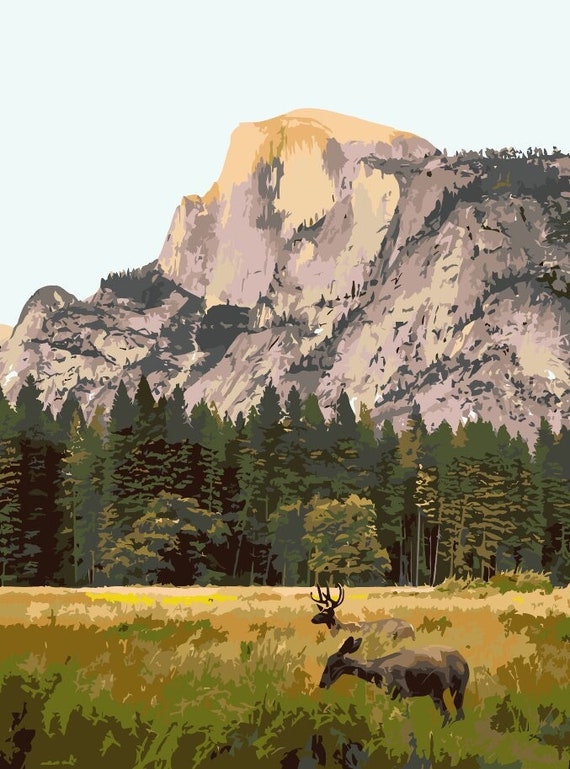This computer-generated image, reminiscent of a painting, features a massive, rocky mountain with a mostly gray, very steep face and patches of greenery sparsely covering about 10-20% of its surface. In the foreground, several tall pine and evergreen trees form a dense cluster, their hues ranging from deep green to lighter shades. Below this tree line stretches a lush grassy field with varying heights and colors: green, yellow, and brown, particularly concentrated towards the front lower left-hand corner. In this serene forest setting, two deer are present; a vigilant buck with prominent antlers stands just a few feet away from a doe, who has large ears and is peacefully grazing. The scene is set under a white sky, enhancing the tranquil beauty of the landscape.